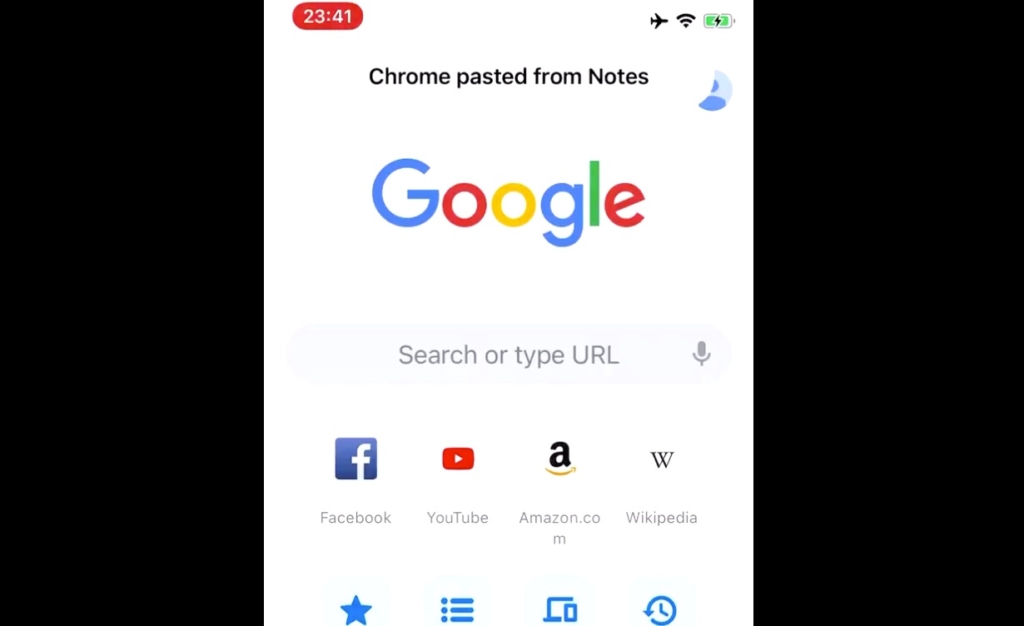The image appears to be a screenshot taken from a smartphone, displaying a web browser interface. Dominating the background is a large black rectangle that frames the screen, with thinner black rectangles flanking the left and right sides. Centrally positioned is a taller white rectangle displaying the phone's interface.

In the top left corner, the time is displayed as 23:41 within a distinctive red oval shape. Moving rightwards along the top, icons indicate that the phone is in airplane mode and connected to Wi-Fi, and the battery icon shows it's charging, represented by a lightning bolt inside a green-filled battery.

Below this status bar, a notification says "Chrome pasted from notes," suggesting recent activity within the browser. The main content area of the screen is taken up by the Google search page, characterized by the iconic multicolored 'Google' logo. The search bar below it includes the prompt "Search or type URL" and features a microphone icon at its right end, indicating voice search capability.

Further down, a row of commonly accessed website icons is visible, including symbols for Facebook, YouTube, Amazon.com, and Wikipedia. Additionally, there are icons for favorites (a star), browsing history (lines), device sync (a computer with a phone), and refresh (a clock).

Overall, this detailed caption captures all the visual elements, making it easy to understand the layout and content of the screenshot.